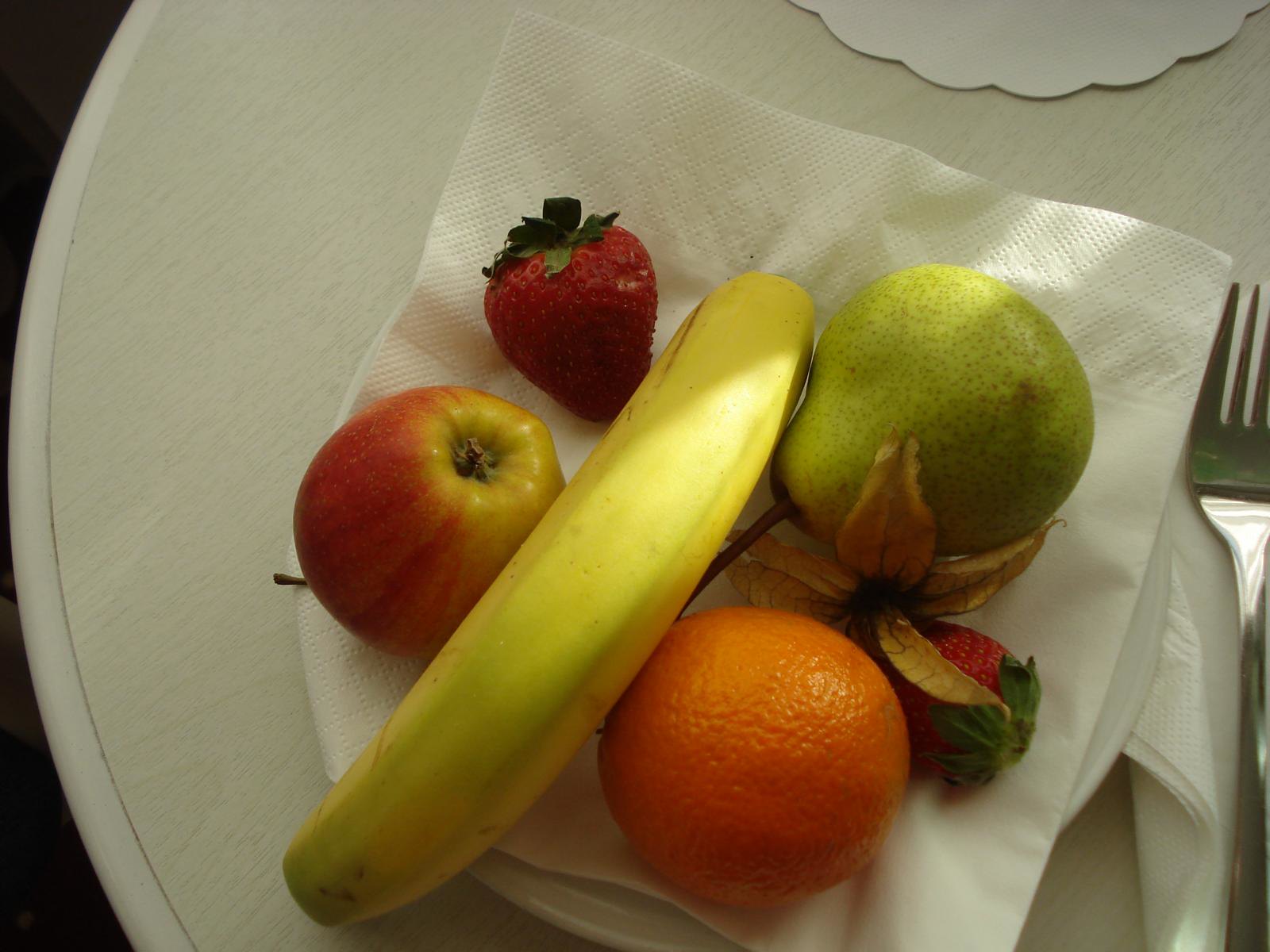Close-up image showcasing a meticulously arranged assortment of fruits on a sleek, flat wide plate. The plate is pristine white and round, providing a clean background that highlights the vivid colors of the fruits. A neatly folded white square paper napkin is positioned centrally on the plate, with a gleaming metal fork placed carefully to the right of the napkin. Resting atop the napkin are six distinct fruits. In the upper left corner, a vibrant red strawberry stands out. Below it, an upside-down apple with a captivating golden brown and red hue grabs attention. Adjacent to these, a large, perfectly ripe yellow banana curves gracefully. Beside the banana, a fresh green pear sits next to another striking red strawberry. Completing the ensemble is a bright orange, adding a final pop of color to the arrangement.